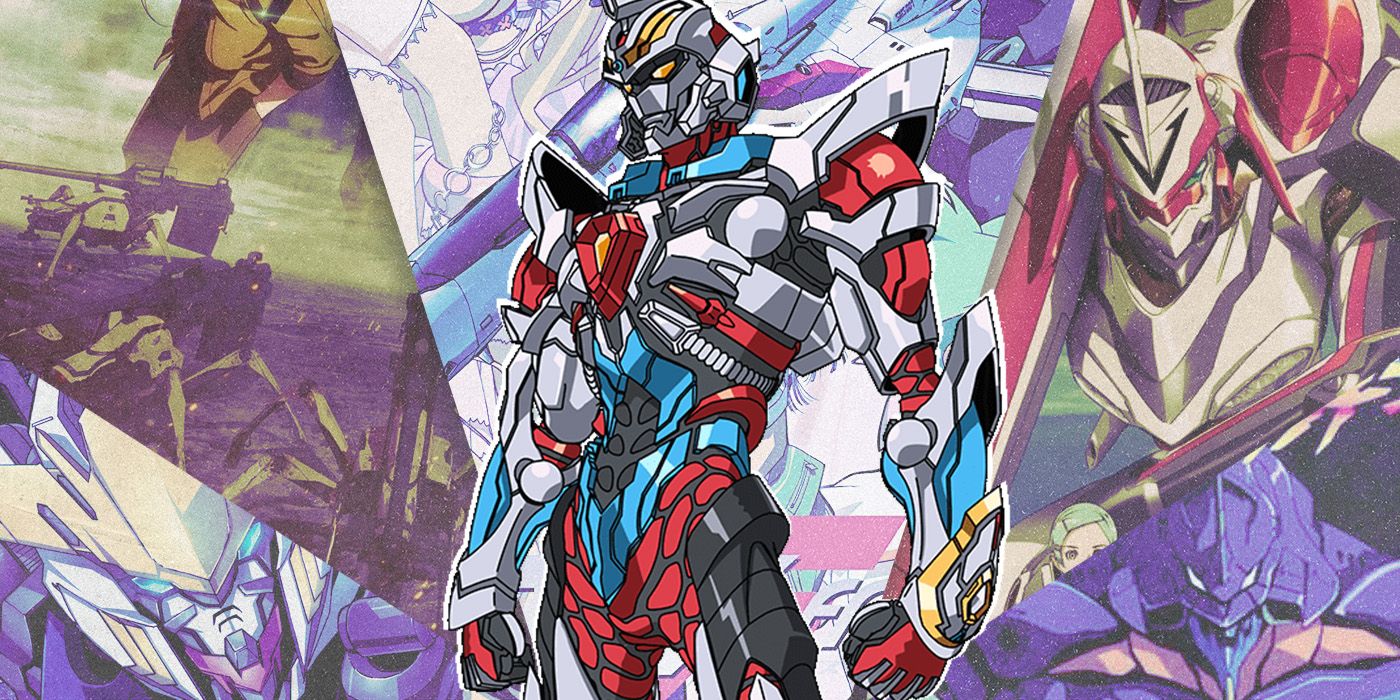In the center of the image is a detailed, humanoid Gundam, standing prominently among various mechs from the same series. The primary Gundam exhibits a sleeker and more humanoid design compared to the typical bulky appearance of mechas, featuring red, yellow, blue, and white prominently in its color scheme. These colors are iconic for the main mecha of the Gundam series. Surrounding this central figure are other mechs that likely inspired this design; notable among them are the classic Gundam in the lower left and a mecha from Neon Genesis Evangelion in the lower right. The background is filled with a vibrant array of other robots, which range in color from purples and greens to oranges and faded reds, creating a colorful and animated scene reminiscent of children's cartoons or movies. This ensemble of mechas makes the setting bright and fantastical, with the central Gundam standing out as the potential leader.